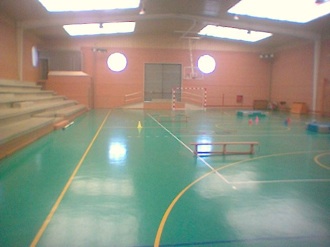The image shows the interior of a multipurpose school gymnasium, characterized by a slightly smoky and hazy atmosphere that renders some details out of focus. The floor of the gym is a bluish-green color, marked with yellow and white lines that delineate playing areas for sports like basketball and possibly indoor soccer. In the center foreground stands a brown bench, while the middle background features a red and white soccer goal with a basketball hoop, complete with a clear glass backboard, situated directly above it.

Towards the far left, there's a row of wooden bleachers, gray in color, likely used for spectators. The back wall of the gym, painted in a reddish-pink or orange hue, includes two large circular windows and a couple of closed doors. The ceiling, adorned with large square lighting fixtures, further illuminates the gym. On the right side of the image, a variety of gym equipment, possibly used for gymnastics and aerobics, is scattered and pushed back, making it somewhat difficult to discern each item clearly.